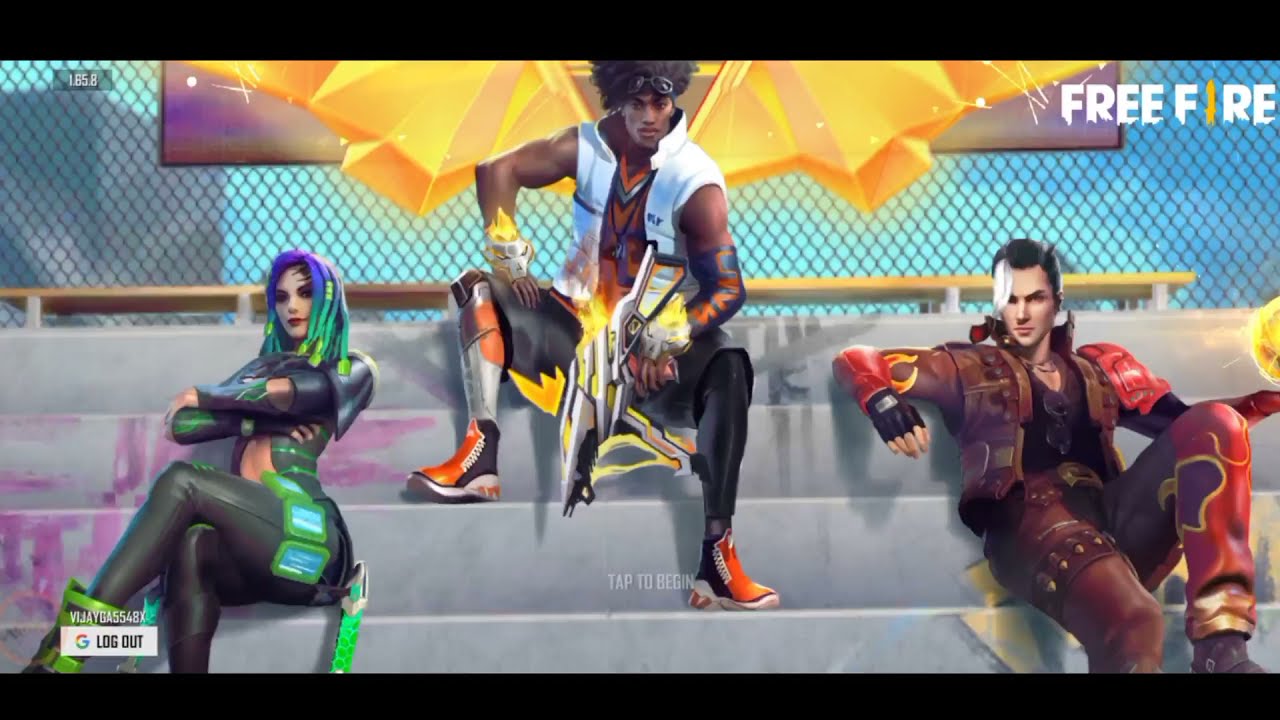The image, which appears to be a screenshot from a video game, depicts three distinct characters sitting on concrete steps that seem to be located outdoors, possibly at the edge of a basketball court. In the background, there's a wire fence against a skyline that includes a skyscraper, suggesting an urban setting. The text "Free Fire" is prominently displayed in the upper right corner, while "Log Out" and "Tap to Begin" are visible in the bottom left and center respectively.

On the right side of the steps is a Caucasian man with black hair, wearing a brown suit over a black shirt, adorned with red armor on his left shoulder, knee, and shin. He wields a white straight cane over his left eye and has flames emerging from his right elbow, with black gloves that expose his fingers. In the center, a black man dressed in a white vest and black pants, equipped with a machine gun, sits on the second step from the top. His shoes are black with orange tops, and his legs are covered in mismatched black and silver cloth. On the bottom left, a woman in a green outfit, sporting blue and green dreadlocks and with her arms crossed, sits with her legs crossed, facing slightly to the left.

This vibrant and detailed scene, rendered in digital art, uses a mix of colors including gray, pink, purple, black, green, orange, yellow, and red, characterized by its stylized, video game aesthetic.